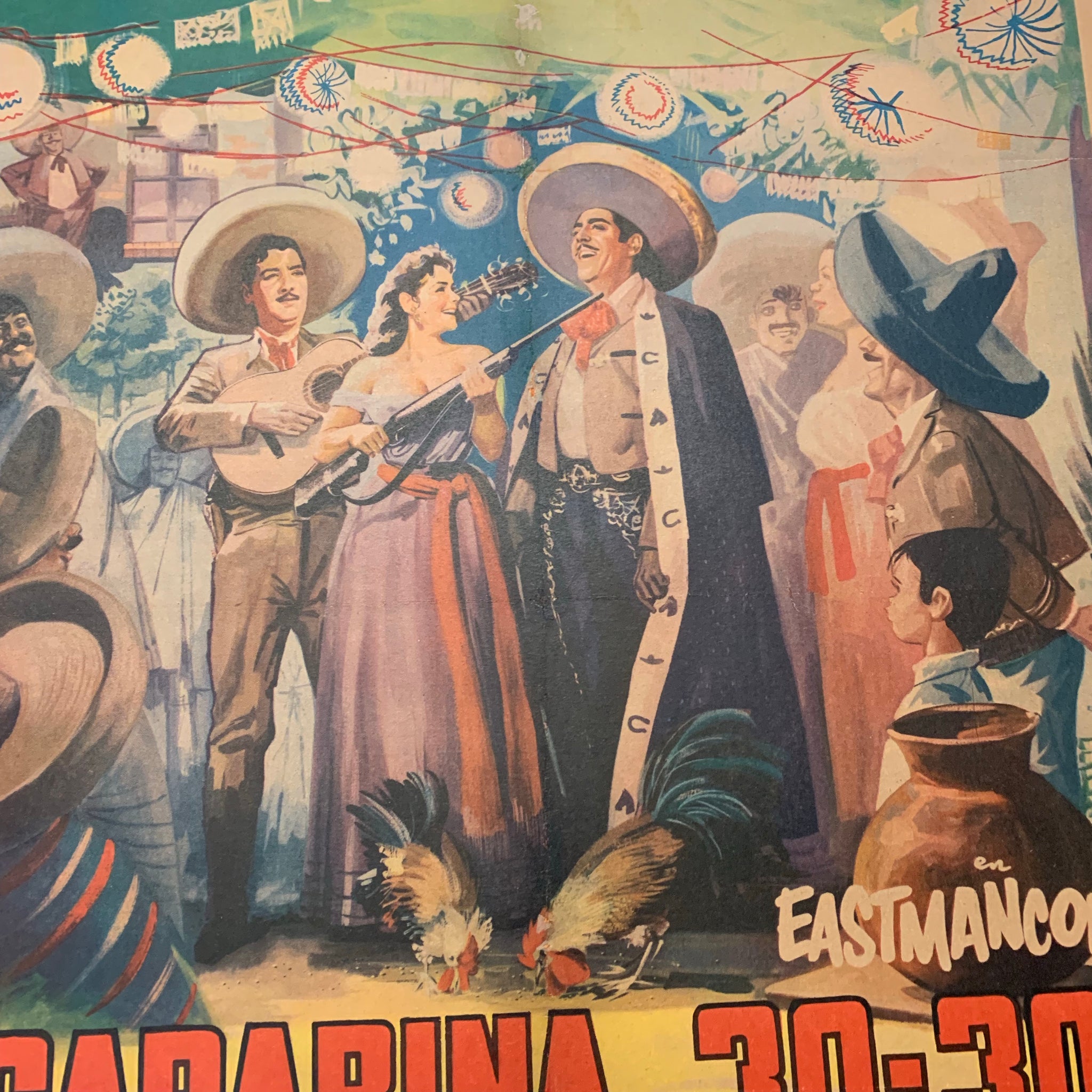The image appears to be a closely-cropped, vintage-style poster, likely for a concert or performance, rendered with pastel, muted colors. It depicts a festive scene suggestive of Mexican or Texan culture, where numerous individuals are adorned in traditional, old Western attire with many sporting sombreros. At the center, a woman wearing a strapless or low-cut dress holds a shotgun towards a man’s throat; both of them are laughing, implying a playful rather than threatening scenario. The man next to her, wearing a long coat or cape, stands nonchalantly. In the background, a third figure, a man with a guitar, is slightly set back but still in focus. At their feet, a couple of chickens or roosters peck at the ground, adding to the rural ambiance. The scene evokes a festive mood, highlighted by decorations and string lights or lanterns overhead, giving the impression of a lively party or festival.